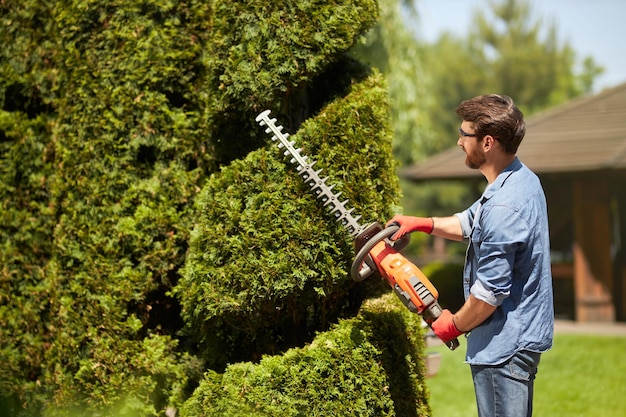In this color photograph taken in landscape mode, we see a man in the foreground meticulously trimming an enormous hedge with an industrial-strength hedge trimmer. The hedge, towering over the man, suggests he's working on a complex topiary design, possibly a circular twist pattern. The man has short dark hair, a beard, and glasses. He is dressed in a blue denim shirt with the sleeves rolled up to his elbows and faded blue jeans. His orange gloves match the hedge trimmer, which has a black serrated blade. Sunlight bathes the scene, casting a shadow of the man and his tool onto the towering greenery. In the blurred background, there is a brown wooden house, some trees, sky, and a bit of grass, adding depth to the setting.